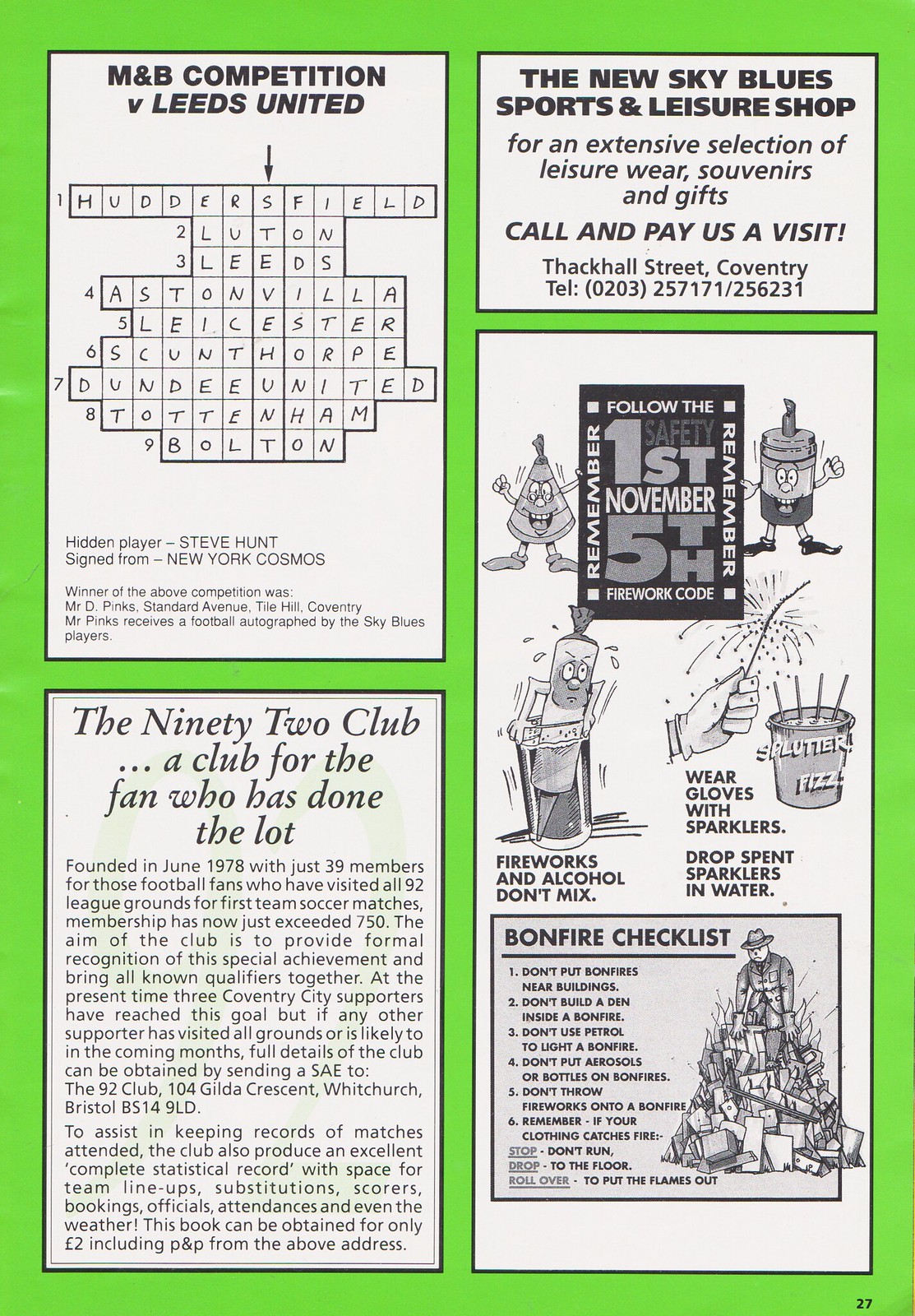The image is an old page from a football club magazine with a lime green background and divided into four white rectangular sections. In the top left, it features an announcement for the "M&B Competition vs Leeds United," accompanied by a word puzzle including terms like Huddersfield, Luton, Leeds, Aston Villa, and others. The hidden player is identified as Steve Hunt, signed from New York Cosmos. Mr. D. Pinks emerged as the competition winner, receiving a football autographed by the Sky Blues Players.

Below this, an article introduces "The 92 Club," a group for football fans who have visited all 92 league grounds. Founded in June 1978 with 39 members, the club's membership has now exceeded 750, recognizing this special achievement and uniting qualifiers. Details on how to join and the club's achievements, including a statistical record book, are also provided.

The top right features an advertisement for the "New Sky Blues Sports and Leisure Shop," offering leisure wear, souvenirs, and gifts, inviting fans to visit their store on Dackhall Street, Coventry.

The bottom right has a bonfire safety checklist, advising on practices like not putting bonfires near buildings, not using petrol, and wearing gloves with sparklers, emphasizing safety during bonfire activities.